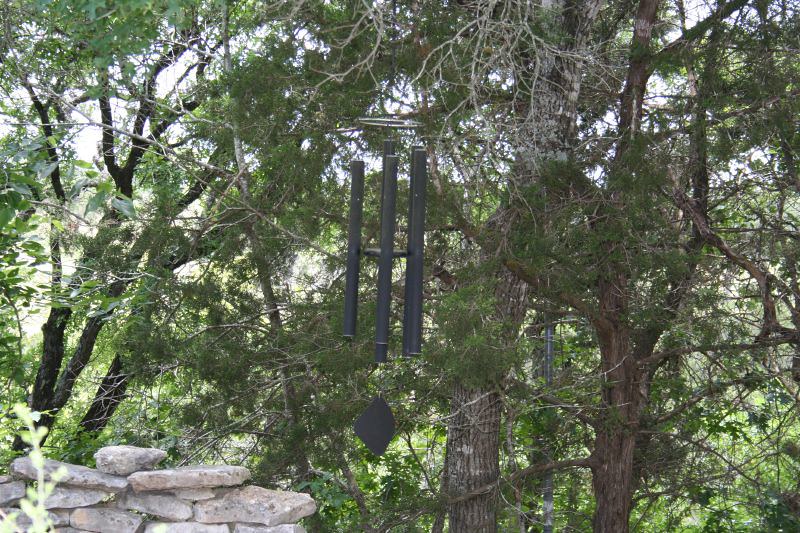In the foreground of this detailed outdoor scene, a large, dark chrome wind chime hangs from a tree. The wind chime features five long, cylindrical bars surrounding a central circular piece, with a flat, black, diamond-shaped clapper hanging from a string in the middle. The top of the wind chime is silver, providing a striking contrast to its darker components. Surrounding the wind chime is a dense wooded area, with a mix of upright and leaning trees. Some trees have leafy branches, while others stand barren. On the left side of the image is a neatly stacked stone wall, composed of white, tan, and pinkish flat rocks, adding an earthy touch to the serene green backdrop. The sky is faintly visible through the dense canopy, completing this tranquil forest scene.